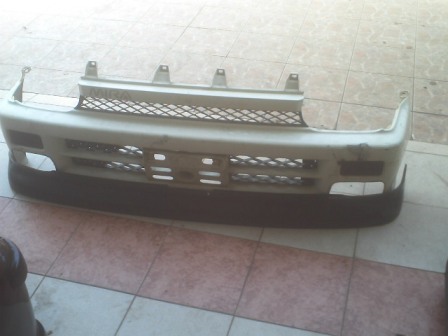In the foreground of the image, there is a white tiled ground featuring a single red-tiled area. Central to the image is a detached bumper from a vehicle, likely a truck due to its larger size. This bumper features a solid black lower portion and a silver section above, which includes a grille area. The bumper has holes for headlights and a designated area for a license plate, suggesting it is made of plastic with spots where it could be bolted to a car. Additional detailing includes what looks like a black object, possibly a fire hydrant or pole, located in the lower left corner. The background features a larger expanse of uniform light gray slate-colored tiles.